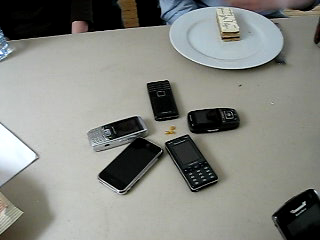The image shows a beige-colored table with five old cell phones arranged in a circle at the center. Among these phones, one is a modern-style touchscreen smartphone while the others are traditional models with small square screens and attached keyboards. Notably, one phone has a silver keyboard while the rest feature black keyboards. Off to the right, there's a round, white plate holding a dessert that appears to be a chocolate treat with white frosting, resembling a custard slice. The people around the table are partially visible; one person's arm in a blue long-sleeve shirt can be seen, as well as another person’s arm wearing a black sweater or jacket. Additionally, a few napkins are placed to the left of the phones, and a partially held-up phone is visible in the foreground.